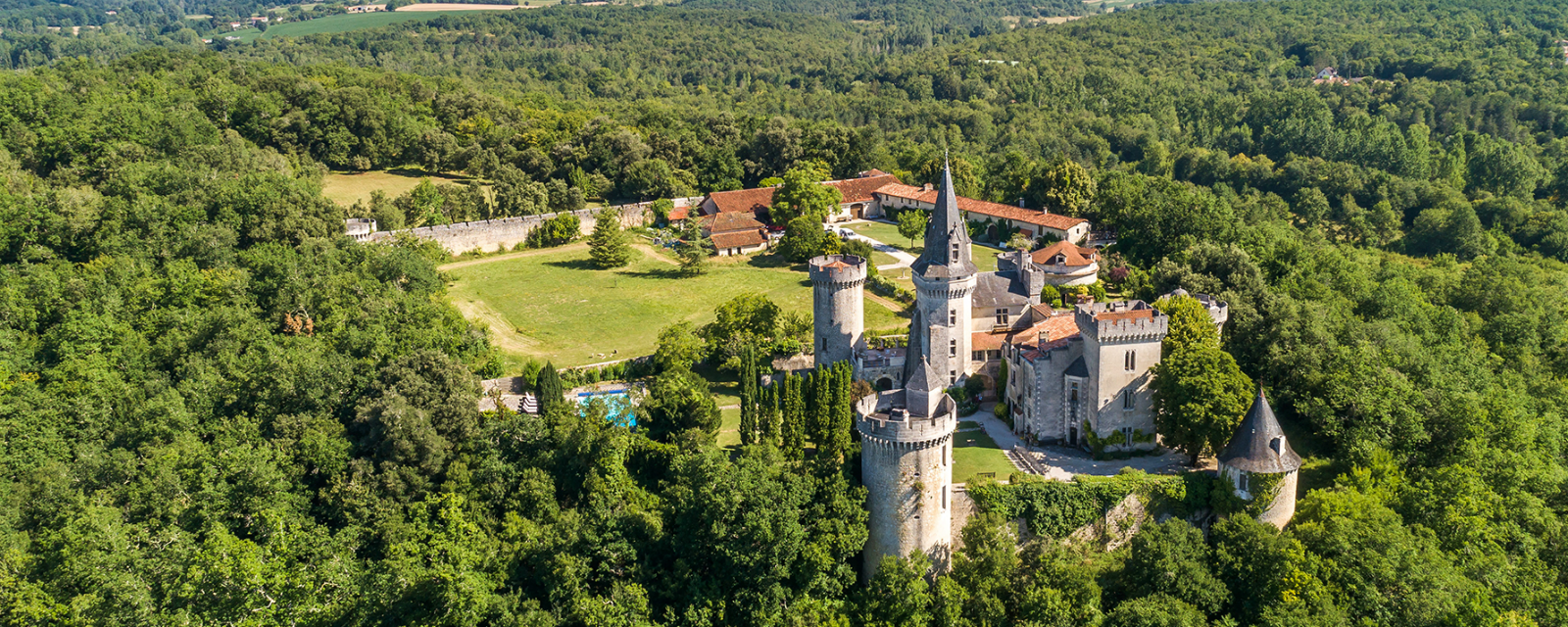This beautifully detailed landscape photograph showcases a magnificent European castle nestled in the heart of an expansive and seemingly endless forest. The forest stretches for miles in every direction, enveloping the castle in a tranquil sea of greenery, creating a secluded and serene atmosphere. The castle, constructed from light gray stone with a brown roof, exudes the charm of a fairy tale, complete with iconic cylindrical towers that evoke images of princesses overlooking their kingdom.

The castle’s extensive courtyard, located behind the main structure, is vast and meticulously maintained. Within this humongous space, which includes neatly trimmed grass and various sidewalks, one can see multiple smaller buildings including regular housing with auburn tile roofs, likely serving as stables or other support structures. There is also a glimpse of what appears to be a small pool, enhancing the sense of luxury and utility within the castle grounds.

In the distant background, beyond the dense forest, there may be hints of farmland, adding to the picturesque and diverse scenery. The entire setting is devoid of human presence or modern vehicles, emphasizing its peaceful isolation and timeless beauty.